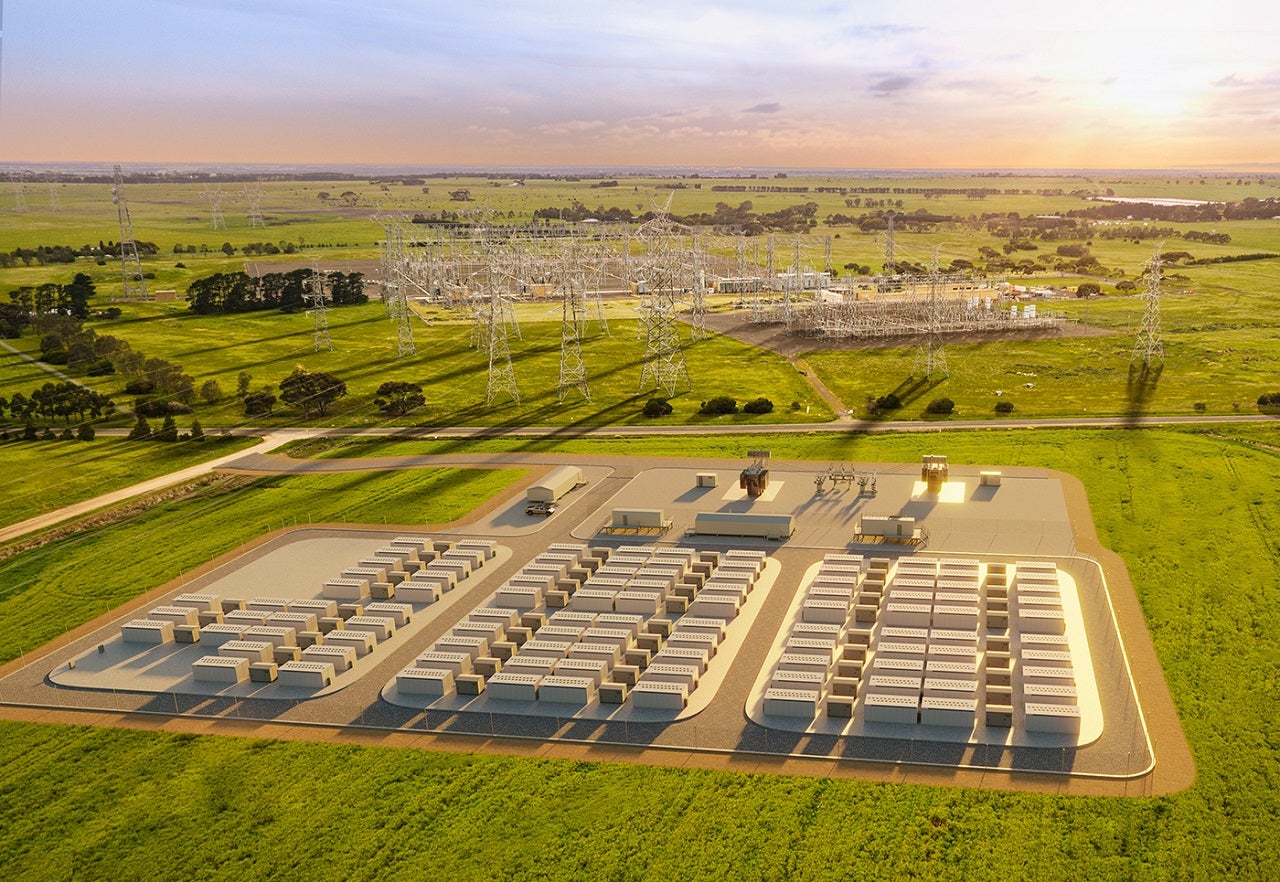This aerial photograph captures a vast, outdoor industrial complex that appears to be a storage facility, possibly for electricity. The landscape is dominated by a large, fenced enclosure filled with a series of aligned, rectangular white structures, which could be buildings or battery storage containers. Surrounding these structures are expansive green fields interspersed with trees and crisscrossed by several roads. In the upper portion of the image, we observe a high-density power substation with numerous metallic poles and power lines casting extended shadows due to the front-facing sunlight. The background showcases a sky adorned with clouds and a striking line of golden hue, indicating an impending sunset. The area is void of human presence or vehicles, emphasizing the scale and isolation of this industrial setting.